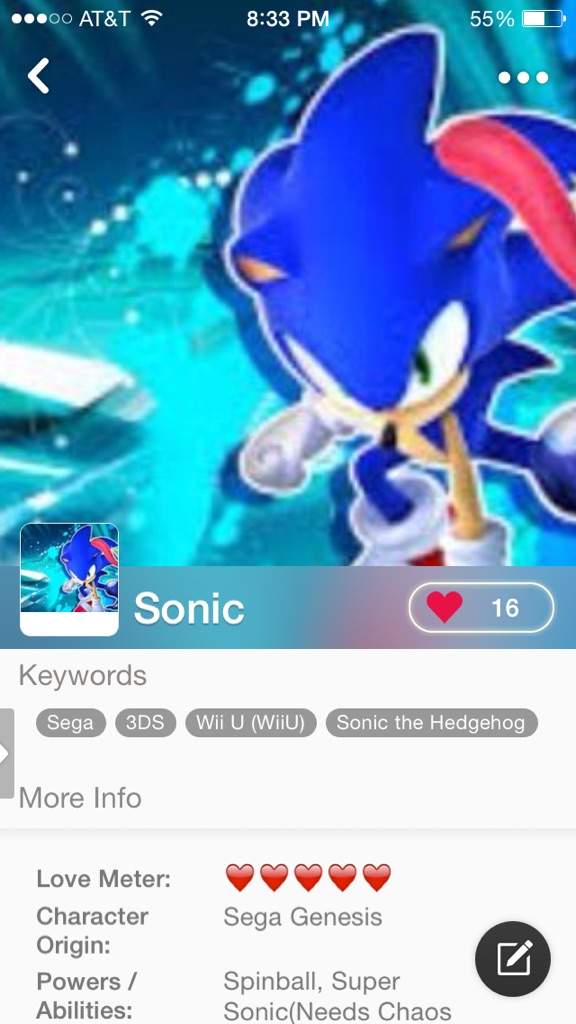A cell phone screenshot displays a Sonic the Hedgehog webpage. In the upper portion of the image, Sonic's blue figure is prominently featured, viewed from above at a downward angle. The character occupies the right side of this section, with a bluish backdrop accentuating his form. Directly below this, there is a navigation bar featuring a smaller, thumbnail version of the main image. To the right of this thumbnail, the word "Sonic" is clearly visible, followed by a heart icon and the number 16, indicating likes or favorites. In the lower section of the screenshot, a white background displays the word "keywords," accompanied by engraved buttons labeled "Sega," "3DS," "Wii U," and "Sonic the Hedgehog."